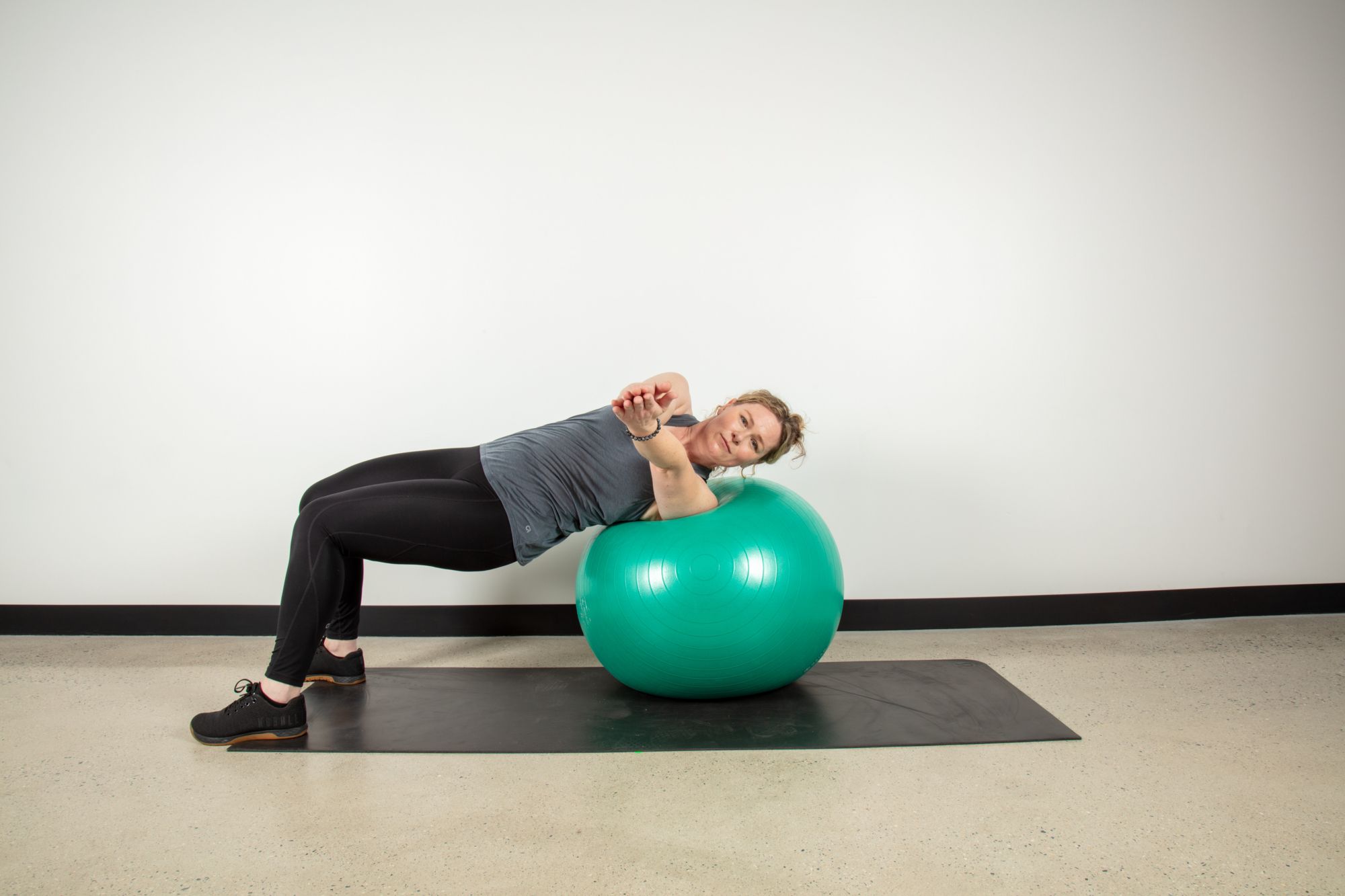In the photograph taken indoors, a woman is seen exercising on a large, turquoise-colored exercise ball. She balances her left shoulder firmly against the ball, her arms extended in a prayer position with her hands flat and pressed down. The woman, who has blonde hair tied back in a ponytail, wears a dark gray tank top, black spandex exercise pants, and black lace-up sneakers without socks. Her legs are extended outward, bent at the knees, and her feet are firmly planted on the beige floor, forming a bridge pattern. She appears concentrated, with her gaze directed straight at the camera. The room features white walls with a black baseboard and is equipped with a black exercise mat underneath the ball.